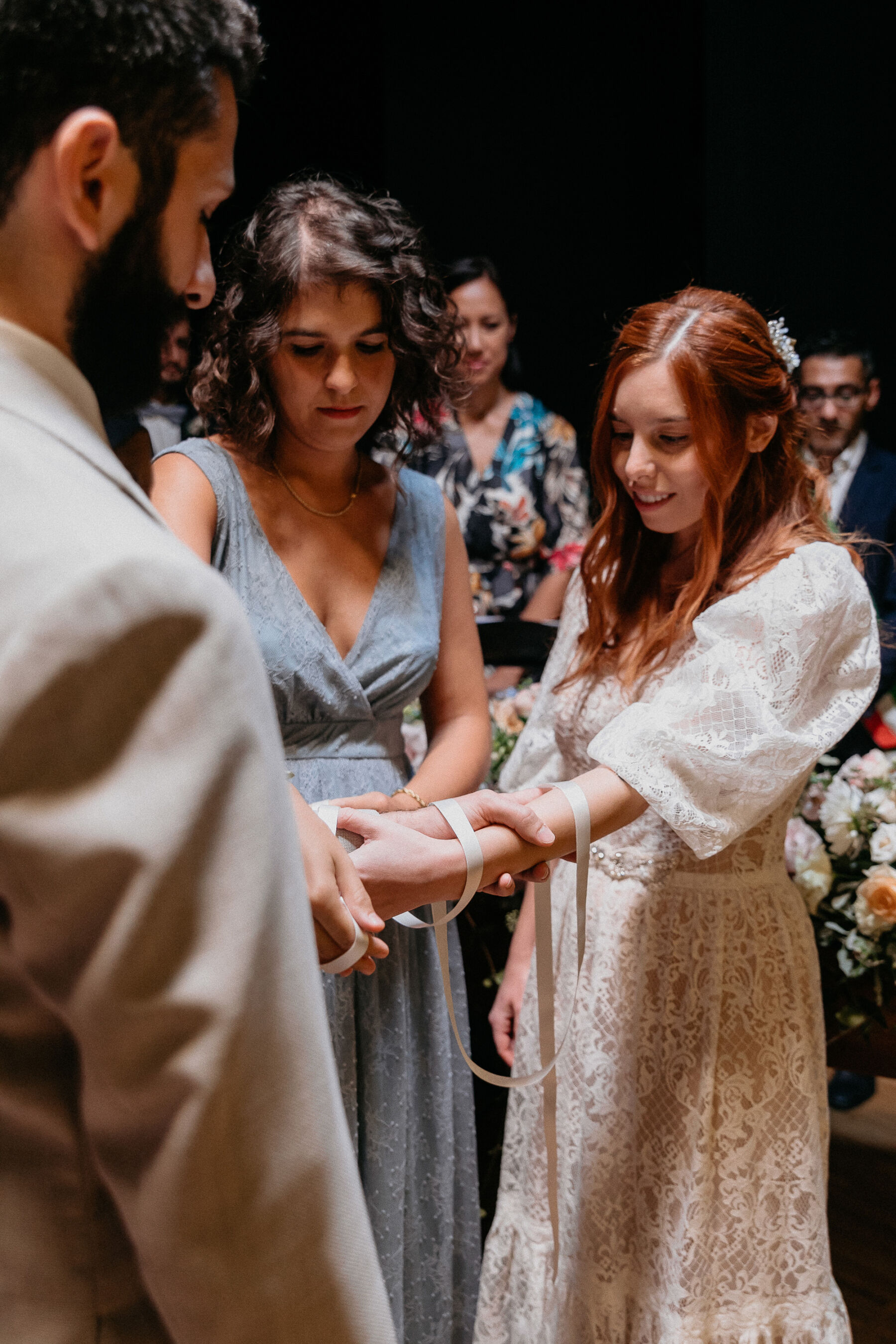This vibrant color photograph captures a unique handfasting ceremony, often associated with pagan and non-traditional wedding rituals. Central to the scene, a dark-haired woman, dressed in a low-cut blue dress, officiates the ceremony. She is carefully wrapping a white ceremonial ribbon around the intertwined wrists of the couple, symbolizing their union. The groom, positioned to the left, sports a full beard and is attired in a light gray suit. The bride, standing to the right, has long, flowing red hair adorned with a small flower behind her ear and wears a simple white dress. The couple's hands are clasped firmly around each other's wrists, emphasizing their bond. Behind the couple, a soft bouquet of flowers adds a picturesque touch, while faintly visible spectators, including both a man and a woman, witness the intimate ritual, contributing to the solemn and harmonious atmosphere of this spiritual union.